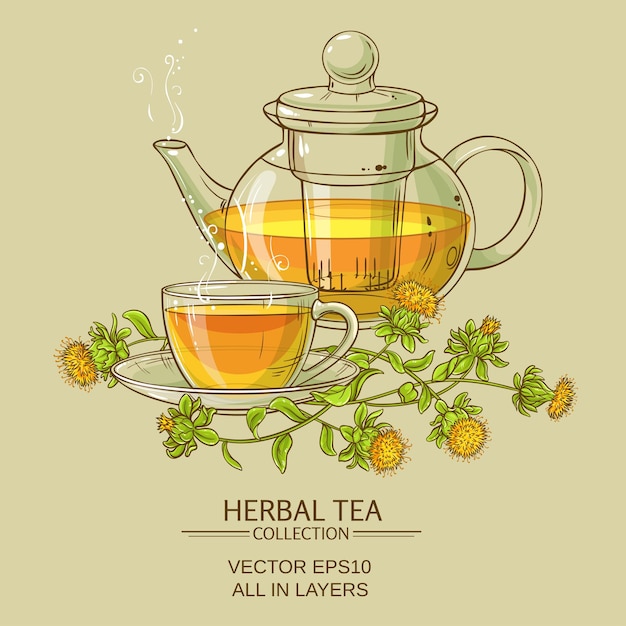The image is a detailed, cartoon-style advertisement for an herbal tea collection. Set against a light tan background, the square image features a clear glass teapot filled with golden-orange herbal tea. The teapot has a visible insert for the tea leaves, a glass handle, and a lid with a large glass knob, with steam rising from its spout. Positioned in front of the teapot is a matching clear glass teacup and saucer, also containing the golden-orange tea. Surrounding the saucer are green stems topped with small yellow flowers. At the bottom of the image, brown text reads "Herbal Tea Collection Vector EPS-10 All in Layers".